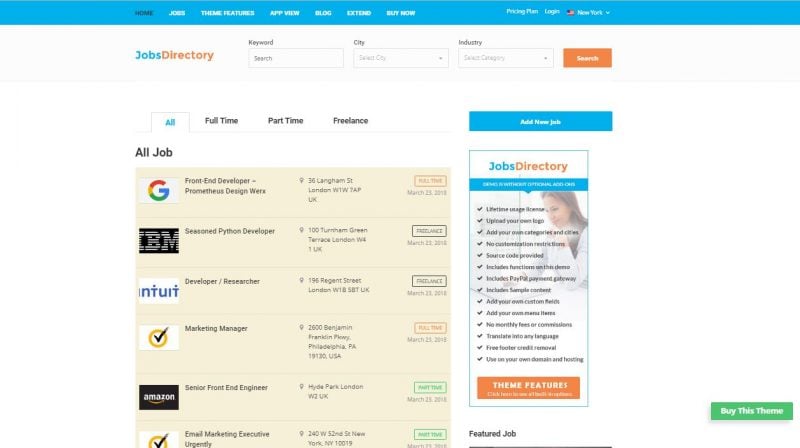The image displays a web page from a job search website called Jobs Directory. The screen is divided into several sections, each serving a specific function. At the top, there is a blue navigation bar with various menu items, although the text appears blurred and undecipherable. Below this, there is a comprehensive keyword search area where users can input job titles, city names, or industries to refine their search results.

The main section of the page is dedicated to displaying job listings. Currently, the filter option is set to "All," which means the viewer is seeing a mix of full-time, part-time, and freelance job opportunities. The job listings are detailed with company names and positions, such as roles at Google, IBM, Intuit, and Amazon. Additionally, there is one entry with the broad title "marketing something."

Each job listing includes an address next to the job title, though the text appears small and challenging to read. On the right-hand side of each listing, there is information indicating the job type (full-time, part-time, or freelance) and the date the job was posted, providing crucial details for prospective job seekers. The interface is reminiscent of other well-known job search platforms like ZipRecruiter, aimed at facilitating efficient job searches for its users.